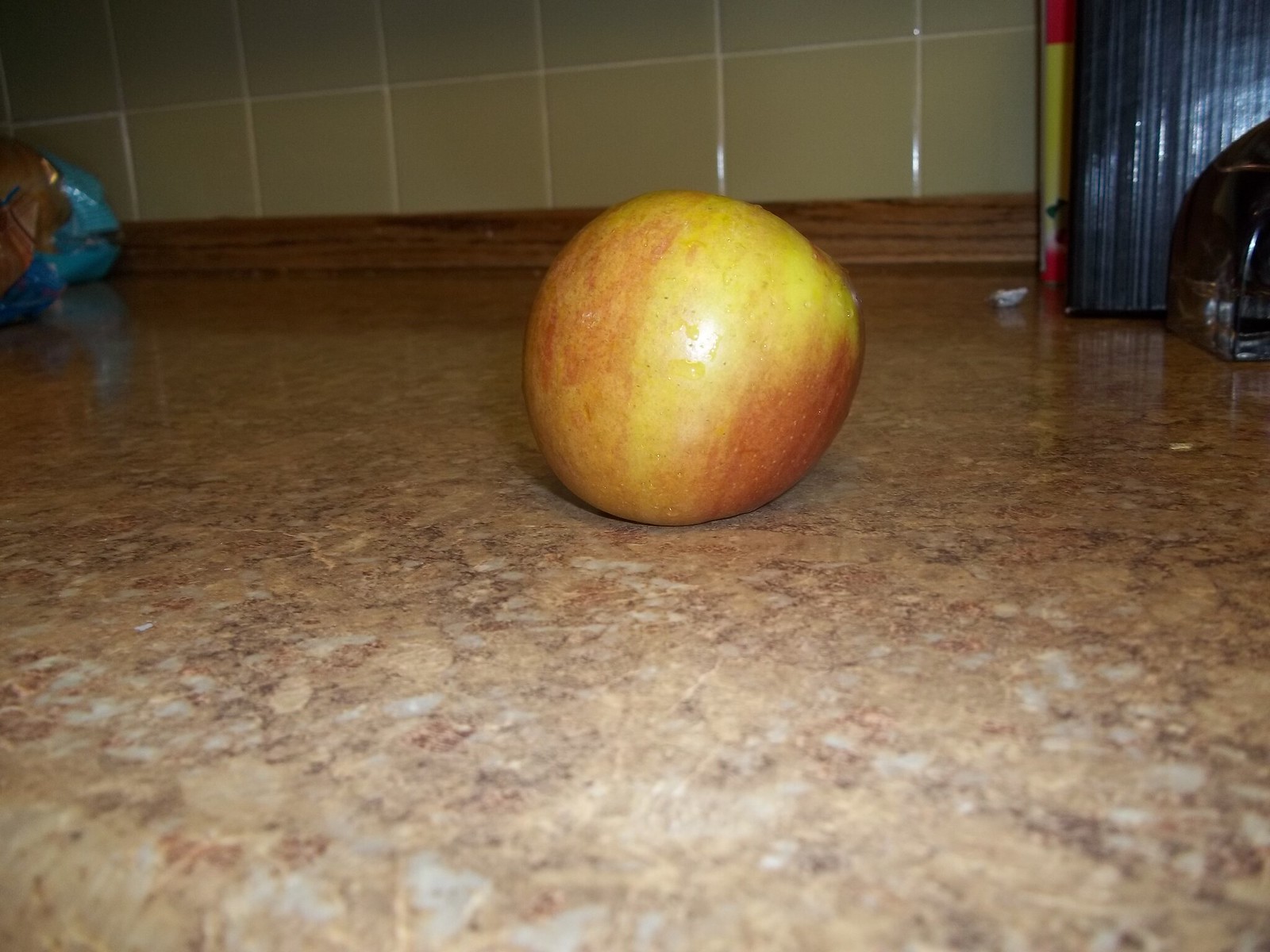In this image, a small, aged apple rests on a marbled kitchen counter. The apple is characterized by a mottled color palette of dark, yellowish hues blending into light reds, especially prominent on its sides. A noticeable light glare at the center hints at the camera's flash. The counter itself showcases a mix of black, light brown, and white tones typical of marble. To the left of the apple, a crumpled light blue plastic package, likely containing bread, is visible. On the right side of the image, a black box or book lies adjacent to a red and yellow surface, with a small black bag propped against it. The kitchen wall in the background features light brown tiles and a wooden baseboard that seamlessly connects the wall to the counter.